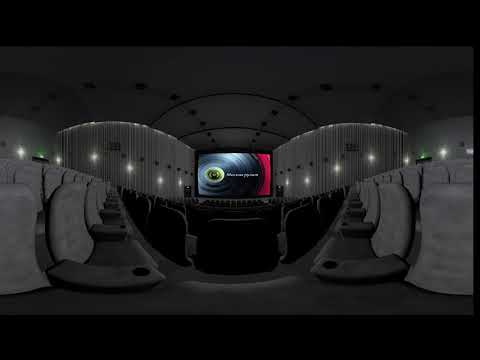This appears to be a panoramic image, possibly a drawing or a 360-degree photograph, of an empty movie theater rendered in virtual reality. In the center of the image sits a very large, rectangular screen displaying a colorful projection with a circular pattern featuring shades of black, white, blue, and red. The movie theater's interior is characterized by rows of grey seats, each with black backs and armrests that include holders for soda cups. The seats ascend in tiered rows, creating a stepped effect. The walls of the theater are white, adorned with LED lights and black background fixtures. The ceiling, also white, displays additional black lighting fixtures. Striated, curtained sections run along the sides of the theater. The overall atmosphere of the image conveys a quiet, empty space.